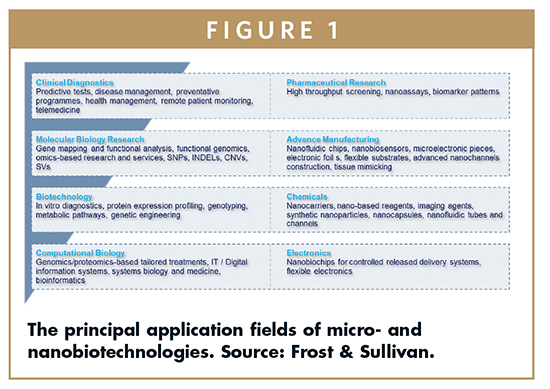This table, typical of those found in scientific journals or articles, presents a visual representation titled "Figure 1," displayed prominently in white font within a rectangular box at the top. Below the title, the table is divided into two distinct columns, each featuring four items, all set against a light blue background. The column titles, written in a medium blue font, clearly differentiate the categories. The table is neatly arranged on a white background, ensuring clarity and readability.

At the bottom of the table, in black font, a description reads: "The principal application fields of micro and nano biotechnologies. Source: Frost and Sullivan."

Within the light blue squares, the detailed entries are as follows:

- **Column 1:**
  1. **Clinical Diagnostics:** Predictive tests, disease management, preventative programs, health management.
  2. **Remote Patient Monitoring:** Telemedicine.
  3. **Molecular Biology Research:** A three-line description.
  4. **Biotechnology:** A two-line description.

- **Column 2:**
  5. **Computational Biology:** A three-line description.
  6. **Pharmaceutical Research:** A one-line description.
  7. **Advanced Manufacturing:** A three-line description.
  8. **Chemicals:** A three-line description.
  9. **Electronics:** A two-line description.

This comprehensive table succinctly encapsulates the various application fields relevant to micro and nano biotechnologies, offering a structured and detailed overview for scientific analysis.